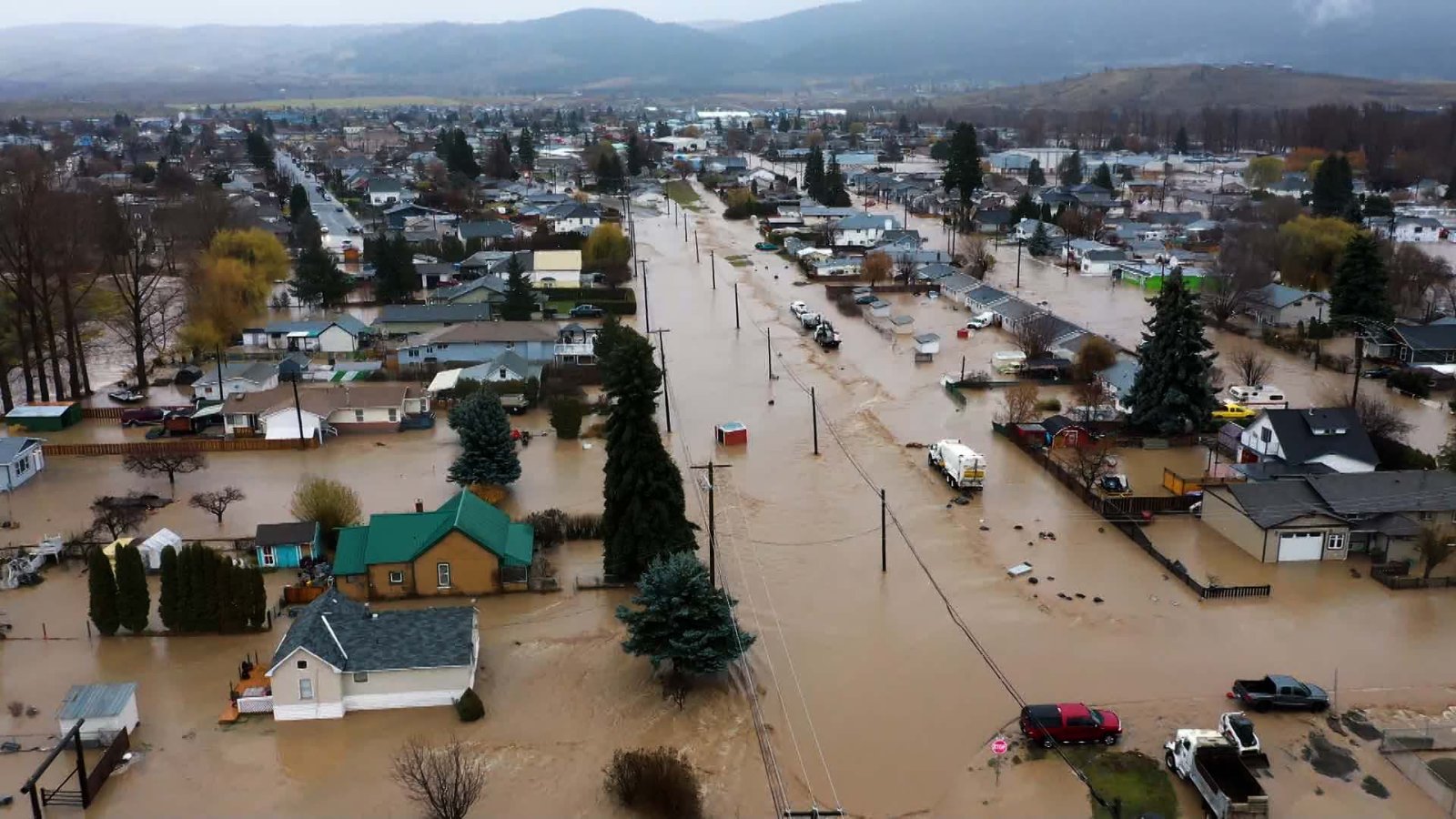This is a detailed bird's-eye view of a sprawling town engulfed in the aftermath of a flood. The image, taken during the daytime, reveals numerous homes and streets inundated with muddy brown water, stretching out as far as the eye can see. The water rises to at least the first level of most buildings, and the entire town appears overwhelmed by the flood. Several vehicles can be seen either driving through the shallow water or parked in it, indicating the flood's depth is substantial but not excessively deep. In the distance, mountains frame the scene on both the left and right sides, adding a somber backdrop to the devastation. The town is densely packed with houses, streets, cars, and other infrastructure, all shrouded in the murky floodwaters, highlighting the extensive impact of the disaster.